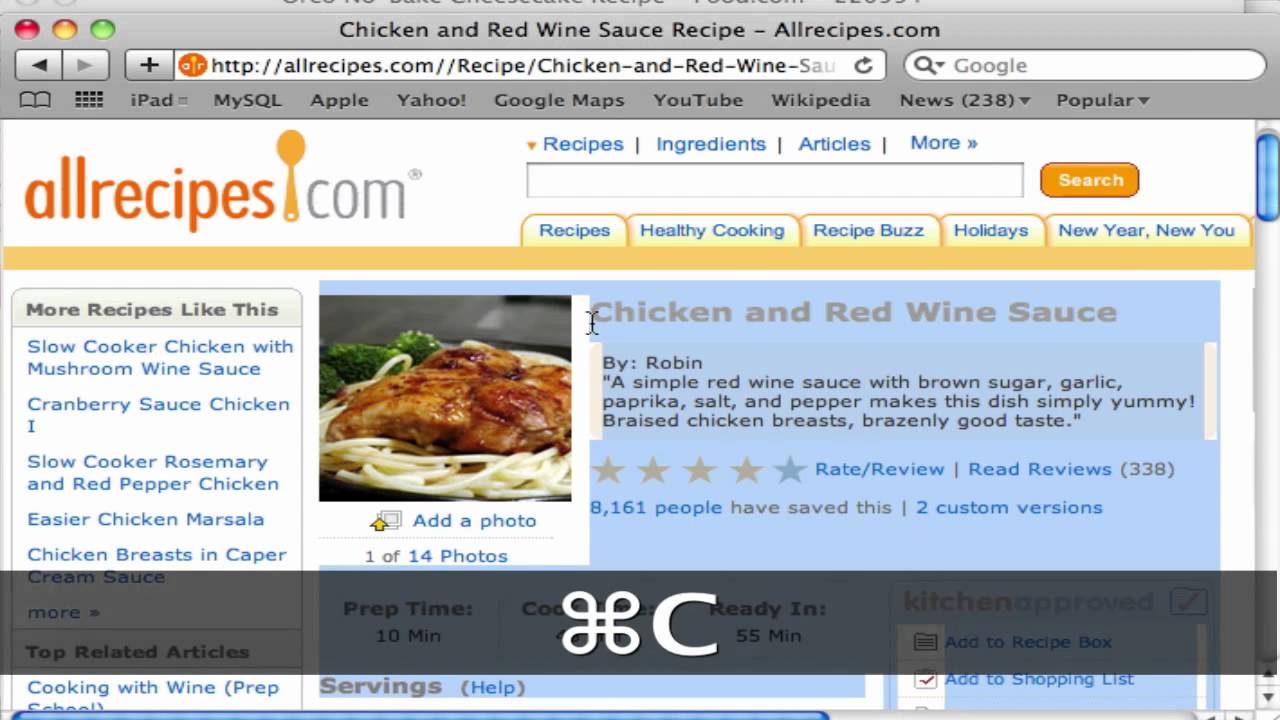A dated screenshot of the Allrecipes.com website displayed on a Mac computer. The web page features the "Chicken and Red Wine Sauce" recipe without revealing the full recipe details in the visible portion of the screenshot. The visible text describes a simple red wine sauce made with ingredients like brown sugar, garlic, paprika, salt, and pepper, highlighting its deliciousness over braised chicken breasts. The website’s interface includes several navigation tabs such as Recipes, Ingredients, Articles, Healthy Cooking, Recipe Buzz, Holidays, New Year, New You, and More Recipes, with additional recommendations listed on the side panel as “More Recipes Like This.”

The recipe has an interactive section showing 338 reviews, with a rating and review option available. There are photos related to the recipe, totaling 14 images. It's noted that 8,161 people have saved this recipe, and it includes two custom versions. The user interface depicted displays typical Apple design elements, including a symbol at the top, the letter "C", and other Mac-specific visual cues, offering a nostalgic glimpse into earlier Apple product designs.